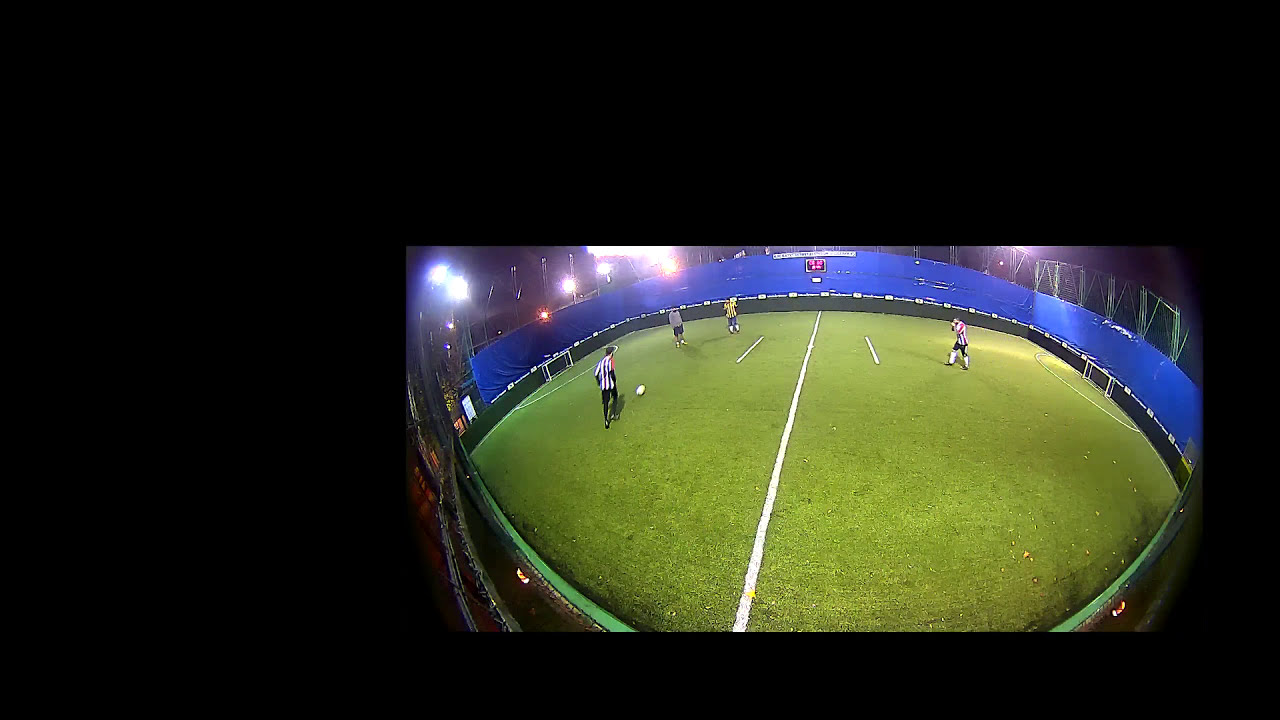This image features a rectangular black background occupying the lower right quadrant, inset with a detailed scene of an indoor soccer field. The prominent half-field midpoint line cuts through the field, which is surrounded by a royal blue perimeter contrasted against the indoor green astroturf. Referees, distinguishable by their black and white vertical striped shirts, are positioned across the field, including one in pursuit of an all-white soccer ball. Notably, the field is illuminated by a cluster of spotlights located towards the left side of the image. Additional players and equipment, including soccer goals at both ends of the field, add to the dynamic athletic setting. The fisheye lens effect curves the edges inward, enhancing the viewer's perspective of this brightly lit nocturnal soccer scene.